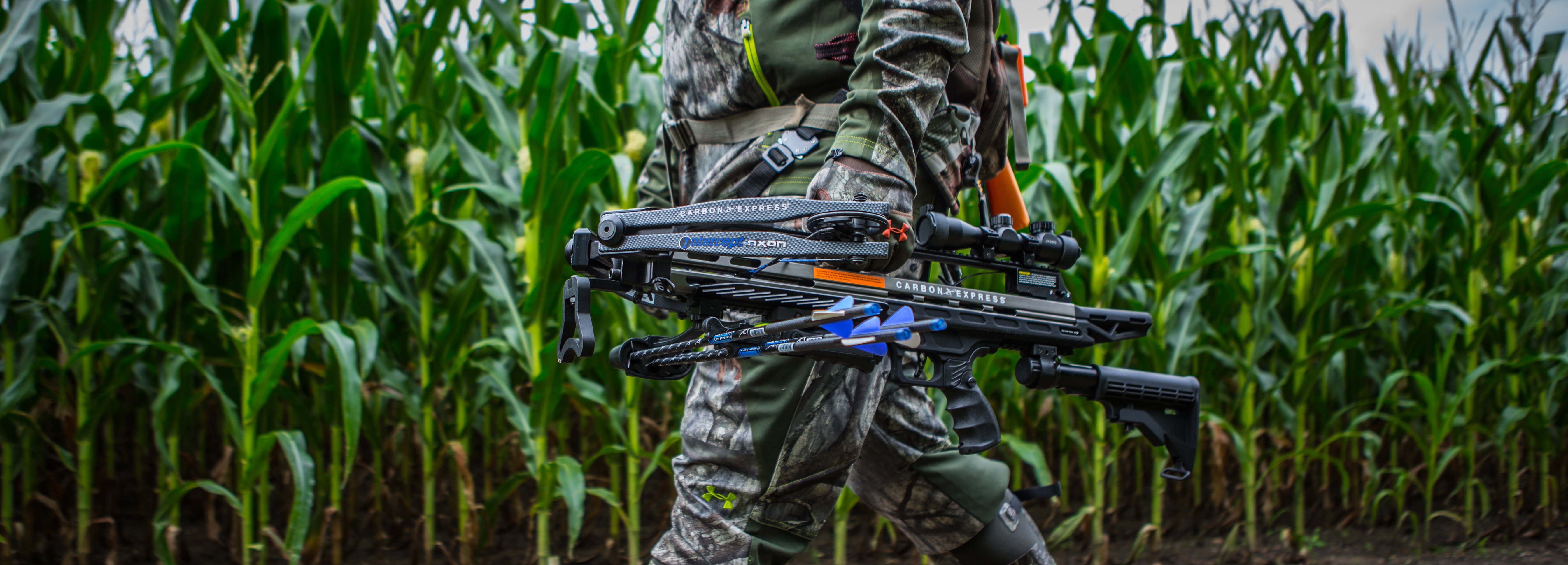A soldier in green and gray camouflage fatigues is walking through a tall cornfield, with green stalks and yellow ears of corn visible behind him. The photo captures him from just above the stomach to his knees, and though details are limited, he appears to be wearing boots. Overcast skies with gray clouds can be faintly seen at the top of the image, suggesting it is daytime. This soldier is heavily equipped, with gear strapped to his back and around his waist. He carries a sophisticated black crossbow featuring various accessories, a scope, a stock, and several bolts with blue fletching secured underneath and attached to it. Some parts of the crossbow have indistinct white and blue text, along with a red bar featuring black text. The crossbow suggests it might be used for hunting.